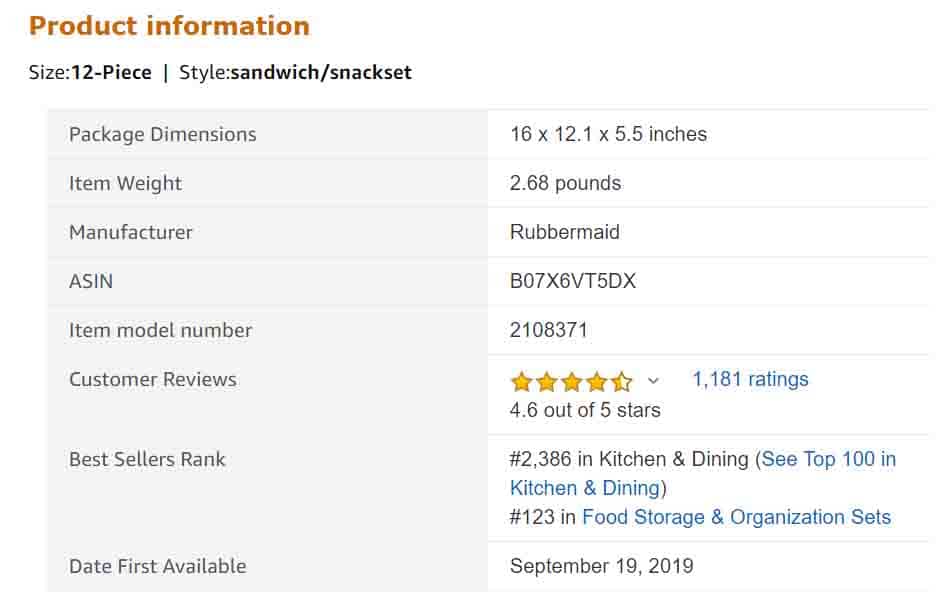This is a photograph capturing product information from an Amazon listing. The image is landscape-oriented and features a predominantly white background, with sections of gray contrast. At the top, the headline "Product Information" is displayed in orange font. Below this header, in black text, are various product details.

The first highlighted item is the size, described as "12-piece" in bold black font. A vertical thin line separates this from the next detail: the style, indicated as "sandwich/snack set" in a darker font.

Following these labels, two distinct boxes appear, each featuring thin horizontal lines that section them into different categories. The left box lists various categories: Package Dimensions, Item Weight, Manufacturer, ASIN, Item Model Number, Customer Reviews, Best Sellers Rank, and Date First Available. 

To the right, corresponding details are provided:
- Package Dimensions: 16 x 12.1 x 5.5 inches
- Item Weight: 2.68 pounds
- Manufacturer: Rubbermaid
- ASIN: [ASIN number not explicitly transcribed]
- Item Model Number: 2108371
- Customer Reviews: 4.6 out of 5 stars based on 1,181 ratings
- Best Sellers Rank: #2,386 in Kitchen and Dining, #123 in Food Storage and Organization Sets
- Date First Available: September 19, 2019

This detailed product info summary is framed against a minimalistic design, focused on delivering essential data in a structured and easy-to-read format.